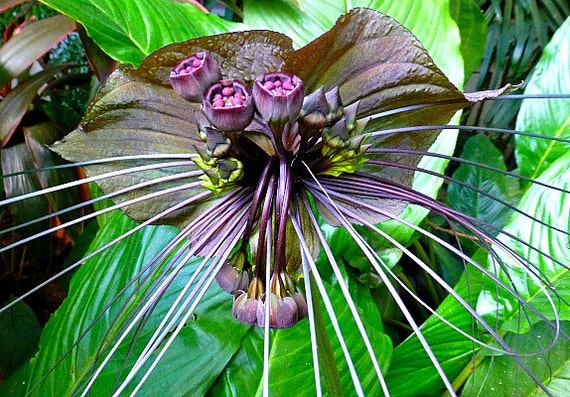This detailed close-up image features an exotic, flowering plant with striking colors and intricate details. The plant's centerpiece displays three prominent, cup-shaped blossoms, each with light purple stamen and pistils, creating a vivid contrast against the petals. These blossoms are surrounded by broad, purplish leaves that have a spade-like shape, meeting in a cluster at the base. Slender, long leaves—25 in total—radiate from this cluster, displaying a mix of green and purple hues that add to the plant's exotic appearance.

To the right of the central blossoms, there are several buds, some ready to bloom and others already opened, revealing their inner beauty. Overlaid against these vibrant flowers are delicate, whispery leaves that extend beyond the petals, adding a dynamic interplay of textures and colors. The background features large, rich green leaves, with some parts revealing thin grass and other plant elements.

In the backdrop, a few out-of-focus plants, possibly palms, contribute to the lush, verdant atmosphere. This setting, combined with dimly lit areas on the left, creates a natural yet mystical ambiance. The overall image captures the elegance and exotic allure of this flowering plant, highlighted by its intricate and colorful details, framed by other lush greenery.